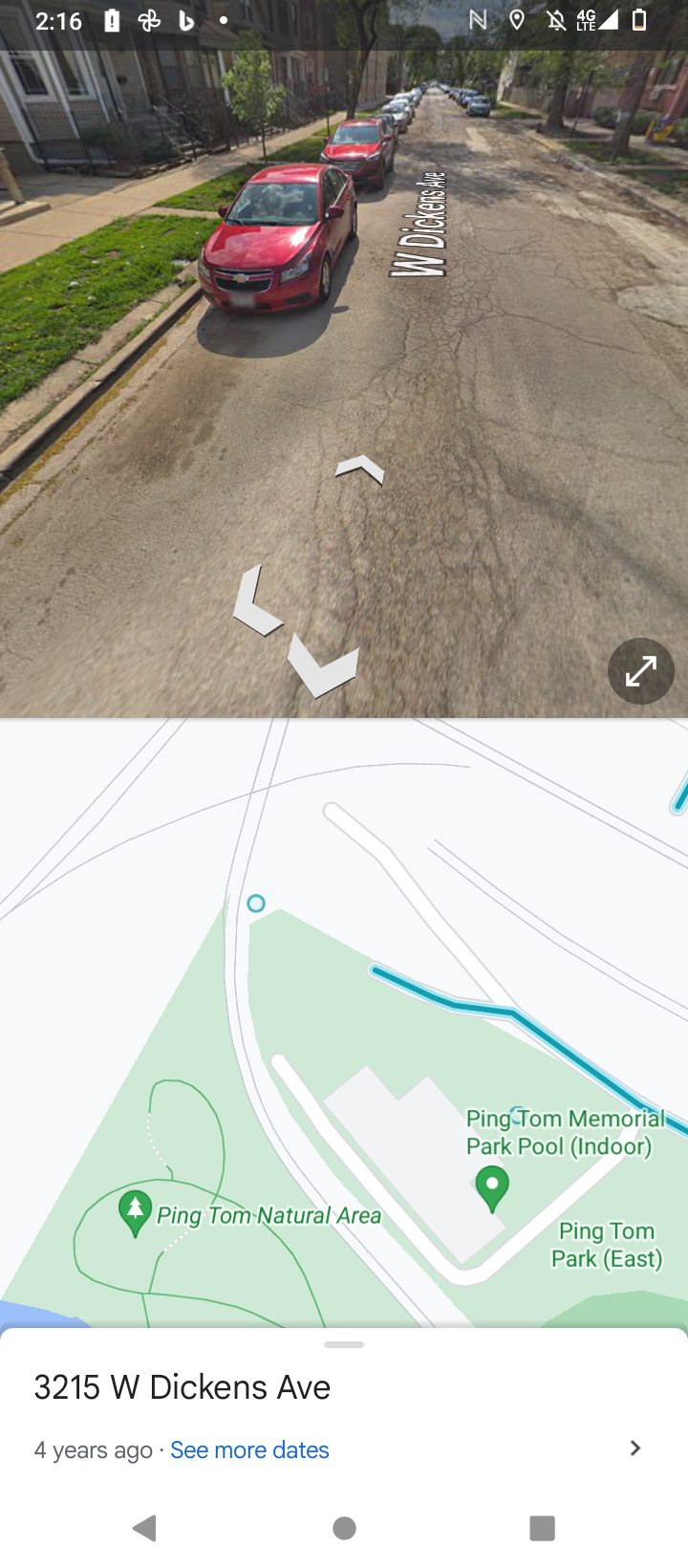This image is a screenshot from a map application, likely Google Maps, as indicated by the status bar at the top showing the time, battery indicator, and other typical smartphone symbols. The primary element is a street view of West Dickens Avenue, with its name displayed in a distinctive, Star Wars-style crawl up the road. Characteristic white arrows for changing the view direction are visible, with an arrow in a circle at the bottom right corner of the photo, signifying rotation.

The street itself is a residential area with notable features: the cracked, frost-heaved pavement, concrete curbs, and green verges separating the sidewalks from the road. Cars line both sides of the street, with two red cars prominently facing the viewer. Trees and several houses are visible, especially on the left side, contributing shade and structure to the scene.

Beneath the street view is an illustrated map of the area surrounding 3215 West Dickens Avenue. The map highlights various streets, a pale green park with specific flagged areas such as Ping Tom Memorial Park, Ping Tom Park East, and a pool, indicating recreational spots. The address "3215 West Dickens Avenue" is printed at the bottom of the image, solidifying the location of this detailed urban snapshot.